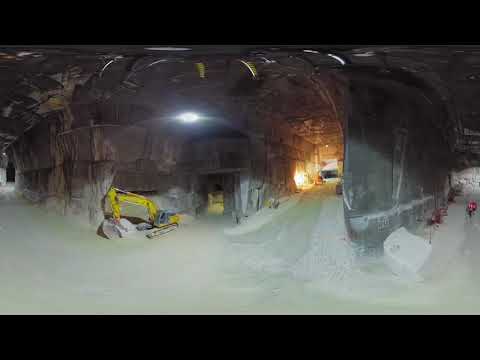This image depicts the interior of a large, industrial underground excavation site, potentially a mine or a salt cave. The passageways of the mine or cave are immense, towering four to five times the height of the yellow excavator visible in the corner. The environment features dusty gravel floors, solid stone walls, and various pieces of industrial equipment scattered throughout. The image presents a panoramic, albeit slightly blurry and low-quality view, possibly from a security camera, which distorts the edges, creating black rectangles at the top and bottom. The ground appears white, possibly covered in salt or ash, adding to the cold and industrial atmosphere.

The lighting within the mine includes a mix of white and yellow-orange work lights, highlighting the various tunnels and passageways. Far off in the distance, you can make out some yellow lights illuminating a rectangular tunnelway that extends deeper into the mine. A large white, cube-shaped stone rests against one of the walls on the right side. The absence of people in the image emphasizes the vast and solitary nature of this underground space.